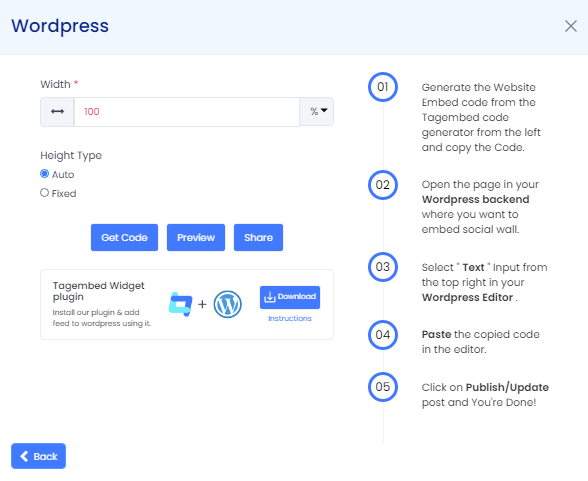This is a color image, seemingly a screenshot of a webpage, with primarily black text on a white background. At the top of the image, there's a light blue rectangle featuring “WordPress” written in blue on the upper left corner and a black 'X' on the right side. Below this header is a box displaying a width with "100" in red positioned in the middle, accompanied by a percentage icon on the right.

Directly underneath, the auto type is selected and highlighted, with "Fixed" positioned below it. Following this section, there are three blue boxes with white text labeled as "Get Code," "Preview," and what appears to be "Shorts," followed by "Share." Another box below mentions the "Tagmented Widget Plugin," with some small, unreadable text beneath it.

Additionally, there’s an image featuring the WordPress icon and another unidentified icon, accompanied by a blue rectangle. Situated at the lower left edge, there’s a blue back button. On the right side of the image, five blue circles are vertically aligned, numbered 01 through 05.

Next to each numbered circle, there's a sequential set of instructions:

1. “Generate the website embed code from this lag embed code generator from the left and copy the code.”
2. “Open the page in your WordPress backend where you want to embed the social wall.”
3. "Select the text input from the top right in your WordPress editor."
4. "Paste the copied code into the editor."
5. "Click on publish/update post, and you’re done."

The image clearly provides a step-by-step guide on embedding content into a WordPress post.